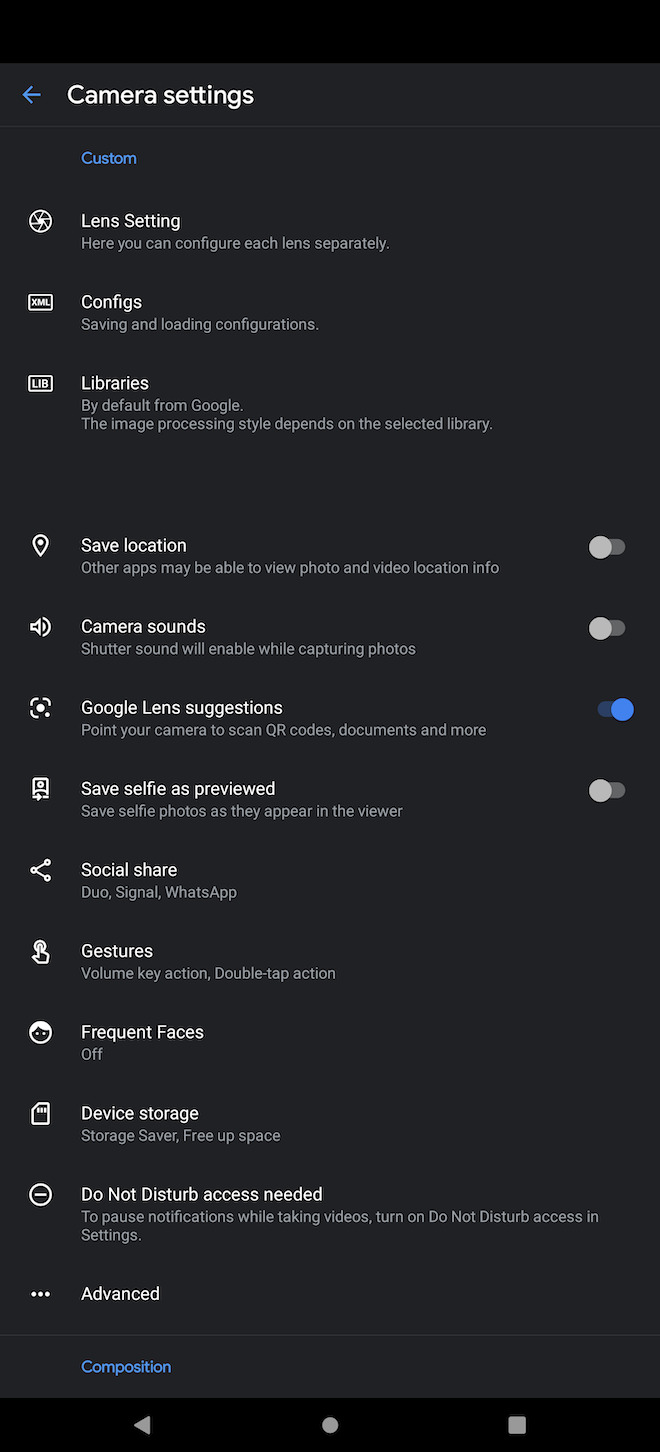Screenshot of Camera Settings Display Detail

The screenshot displays an extensive view of camera settings, delineated into various categories and options:

- **Navigation and General Settings**: 
  - **Top Left**: A blue arrow icon points to the left, facilitating the return to the previous screen.
  - **Header**: The title "Camera Settings" appears, with the subtitle “Custom” in small blue letters below it. 

- **Lens Setting**:
  - **Label**: "Lens Setting"
  - **Description**: Indicates "Here you can continue each lens separately."

- **Configuration Options**:
  - **Config Saving and Loading**: Options for saving and loading configurations.
  - **Libraries**: Details that by default, Google’s image processing style depends on the selected library.

- **Save Location**:
  - **Toggle**: An on/off switch displayed, currently set to off.
  - **Note**: Mentions that other apps may view video location information.

- **Camera Sounds**:
  - **Status**: Turned off.
  - **Details**: Shutter sound will enable while capturing photos.

- **Google Lens Suggestions**:
  - **Toggle**: Turned on, indicated by a blue button positioned to the right.
  - **Details**: Suggests pointing the camera to scan QR codes, barcodes, documents, and more.

- **Save Selfies as Previewed**:
  - **Toggle**: Allows saving selfies exactly as previewed, currently turned off.

- **Social Share**:
  - **Services**: Includes options for Duo, Signal, and WhatsApp.

- **Gestures**:
  - **Details**: Describes available gesture actions, such as volume key action and double-tap actions.

- **Frequent Faces**:
  - **Status**: Turned off.

- **Device Storage**:
  - **Details**: Options for managing device storage, including storage server and free up space.

- **Do Not Disturb Access Needed**:
  - **Note**: Indicates that to pause notifications while taking videos, users need to enable Do Not Disturb access in settings.

- **Advanced Options**: 
  - **Indicator**: Signified by three dots.
  - **Composition**: Displayed in small blue letters with an arrow pointing to the left, and a centered gray square-in-circle icon.

This detailed reference comprehensively captures each setting and its functionality within the camera's configuration interface.